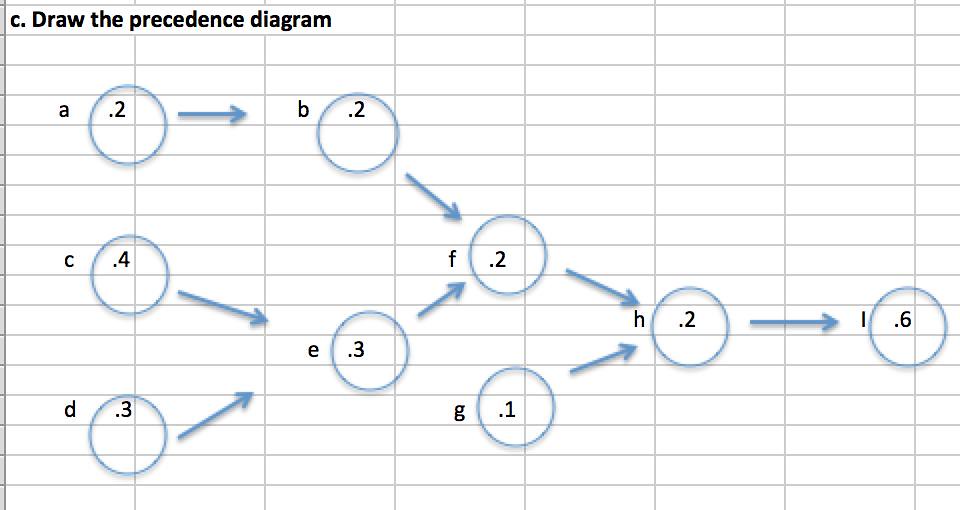The image features a hand-drawn diagram on lined paper designed to resemble a Google Doc or Google Worksheet. At the top of the page, the text reads "C. Draw the precedence diagram," spanning three equal-width columns.

The diagram itself is an intricate network of nodes and arrows, organized as follows:

1. Node A (labeled as 0.2) is connected by an arrow pointing to Node B.
2. Node B (labeled as 0.2) branches out with arrows leading to Node C (0.4) and Node D (0.3).
3. Node C (0.4) further branches down to Node E (0.3).
4. Node E (0.3) connects up to Node F (0.2).
5. Node F (0.2) branches off to Node G (0.1) through a downward arrow.
6. Node G (0.1) is linked to Node I (0.6) by an ascending arrow.

This structured layout, featuring columns and nodes interconnected by directional arrows, serves to illustrate complex relationships in a clear and methodical manner.